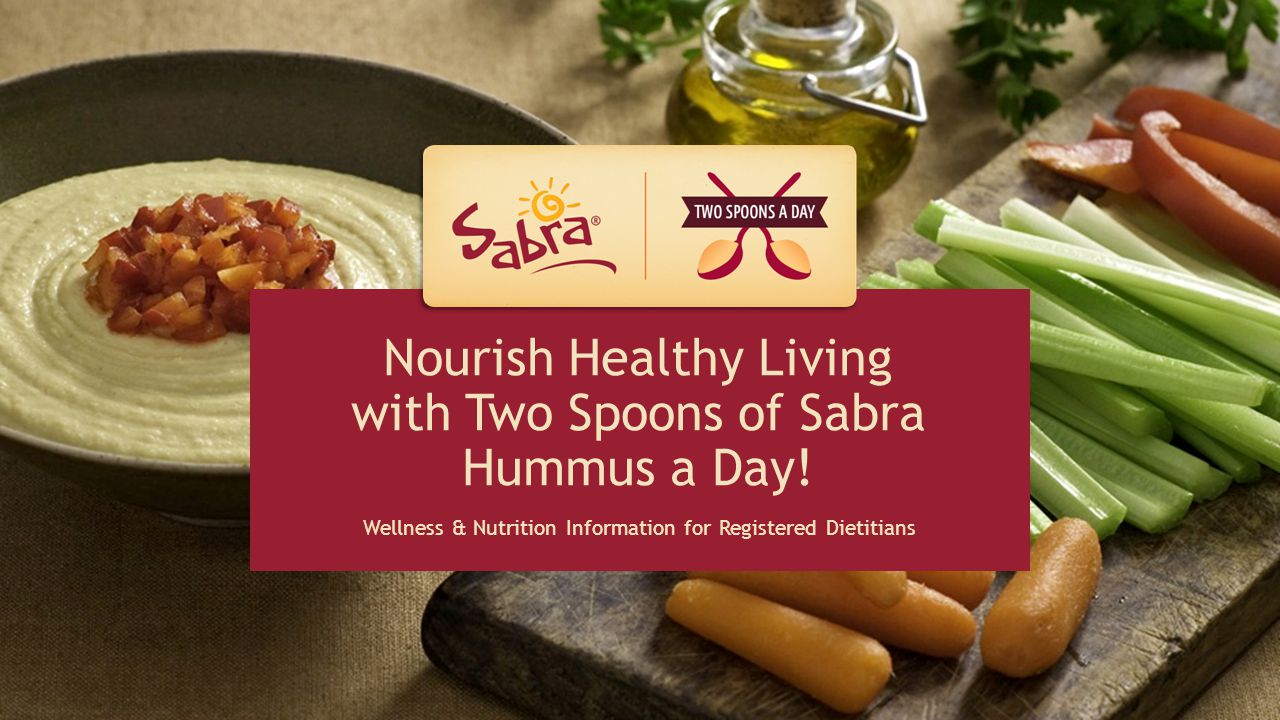The advertisement showcases a beautifully styled food scene centered around a bowl of hummus, highlighted by the text "Sabra, Two Spoons a Day" in the middle. The bowl, a dark black color, contains almost white hummus, garnished in the center with finely chopped brown bits. Complementing the hummus, to the right, is a wooden cutting board featuring an assortment of fresh vegetables, including green celery and red bell peppers. Above these, on the top center of the image, is a jar of olive oil, with sprigs of parsley peeking from the corner. The cutting board's rich dark brown color complements the earthy tones of the hummus and vegetables. The text, placed against a maroon background, is accompanied by a bright yellow sun logo above the word "Sabra." It reads: "Nourish healthy living with two spoons of Sabra hummus a day. Wellness and nutrition information for registered dietitians." The setting elegantly merges elements of freshness and health, inviting viewers to integrate Sabra hummus into their daily diet.